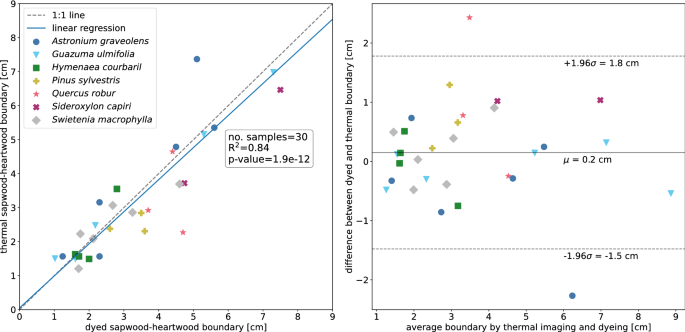The image features two side-by-side scatter plots depicting the relationship and differences between the thermal and dyed sapwood-heartwood boundaries in various tree species. The left graph has the y-axis labeled "Thermal Sapwood-Heartwood Boundary (CM)" and the x-axis labeled "Dyed Sapwood-Heartwood Boundary (CM)." Data points representing different species are plotted, with a blue linear regression line indicating a positive correlation from the bottom left to the top right. The legend identifies species with various markers: blue circle for Astronium Graveolens, blue triangle for Guazuma Ulmifolia, green square for Hymenaea Courbaril, yellow plus sign for Pinus spp., pink star for Quercus spp., pink X, and gray diamond.

The right graph examines the difference between dyed and thermal boundaries against the average boundary obtained from thermal imaging and dyeing. The y-axis is labeled "Difference between Dyed and Thermal Boundary (CM)," and the x-axis is labeled "Average Boundary by Thermal Imaging and Dyeing (CM)." This plot displays scattered points without a clear correlation, with most species' data points ranging between 1 to 4 on one axis and -1 to 1 on the other. Both plots provide insight into the relationship and discrepancies between measuring techniques across different species.